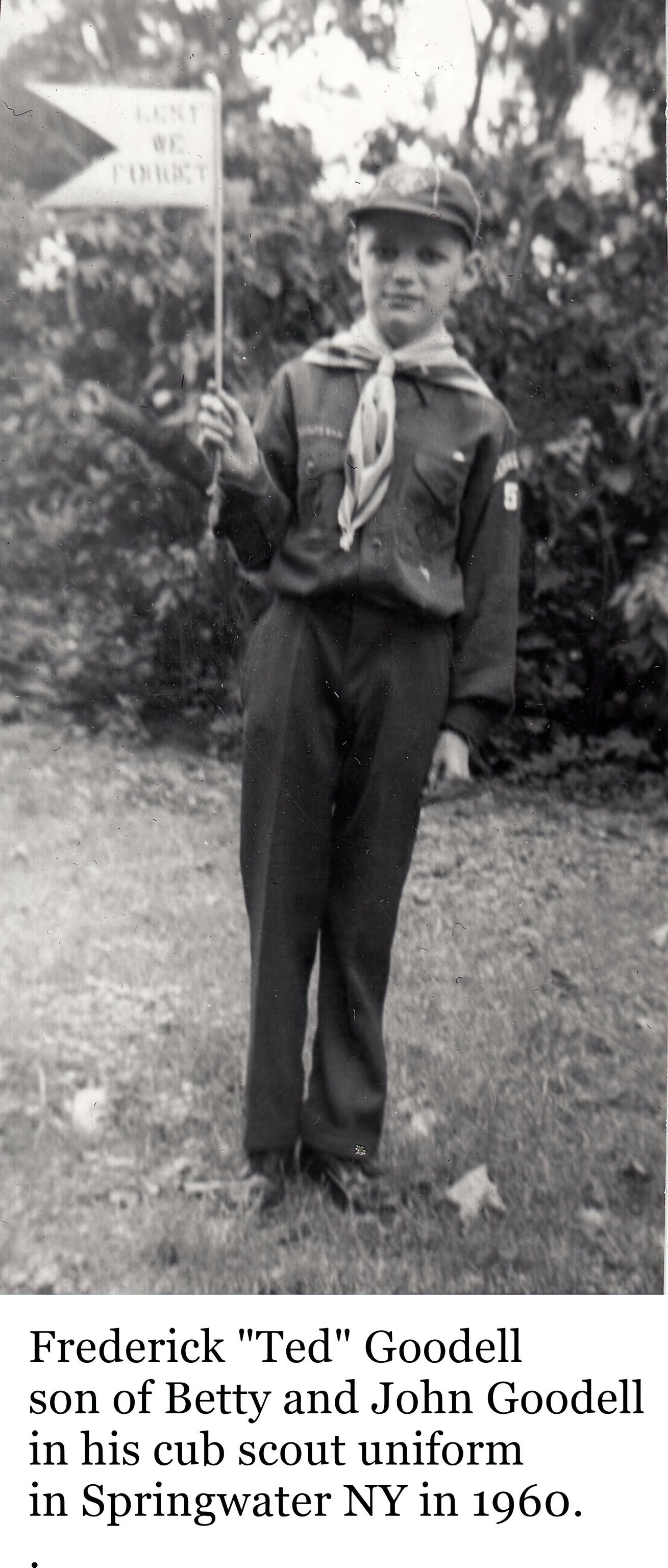This is a detailed black and white photograph from 1960 featuring a young Frederick Ted Goodell, son of Betty and John Goodell, dressed in his Cub Scout uniform. Frederick stands proudly on a grassy area, possibly a park or his backyard, holding a flag with text on it in his right hand. The pennant mounted on a thin stick, points to the left. He wears long pants, a long-sleeved shirt, a scarf around his neck, and a baseball cap on his head. Behind him, tall bushes frame the scene with glimpses of the sky peeking through, and a few fallen leaves scattered at his feet suggest it's either late summer or early fall.